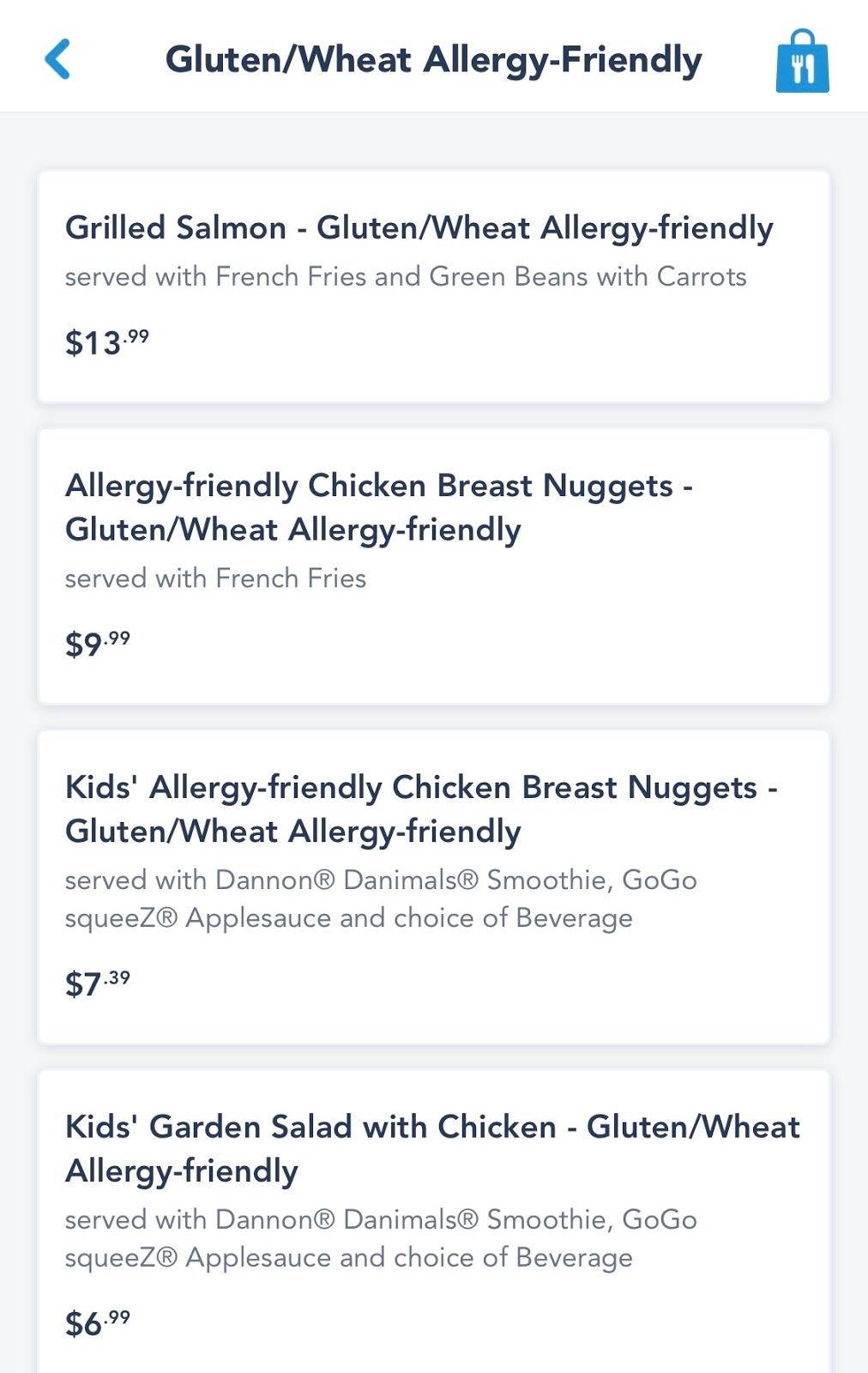A screenshot of a mobile application displays various gluten and wheat allergy-friendly meal options. 

In the upper left corner, there is a blue arrow pointing left, which serves as a back button. Next to it, the text reads "Gluten/Wheat Allergy-Friendly." Just to the right, there is an icon of a bag with a fork and knife on it. 

The first item listed is "Grilled Salmon - Gluten/Wheat Allergy-Friendly," priced at $13.99. This dish is served with French fries and green beans with carrots.

The second item is "Allergy-Friendly Chicken Breast Nuggets - Gluten/Wheat Allergy-Friendly," priced at $9.99 and served with French fries.

Next, there is an option for "Kid's Allergy-Friendly Chicken Breast Nuggets - Gluten/Wheat Allergy-Friendly," priced at $7.39. This meal is accompanied by a small serving of Tannini or Tannini Emuls Smoothie and GoGo squeeZ applesauce, along with a choice of beverage.

The final item is another kid's meal, labeled "Kid's Allergy-Friendly - Gluten/Wheat Allergy-Friendly," priced at $6.99. This meal is also served with Tannini or Tannini Emuls Smoothie, GoGo squeeZ applesauce, and a choice of beverage.

The detailed information presented offers a comprehensive guide to gluten and wheat allergy-friendly options available in the app.